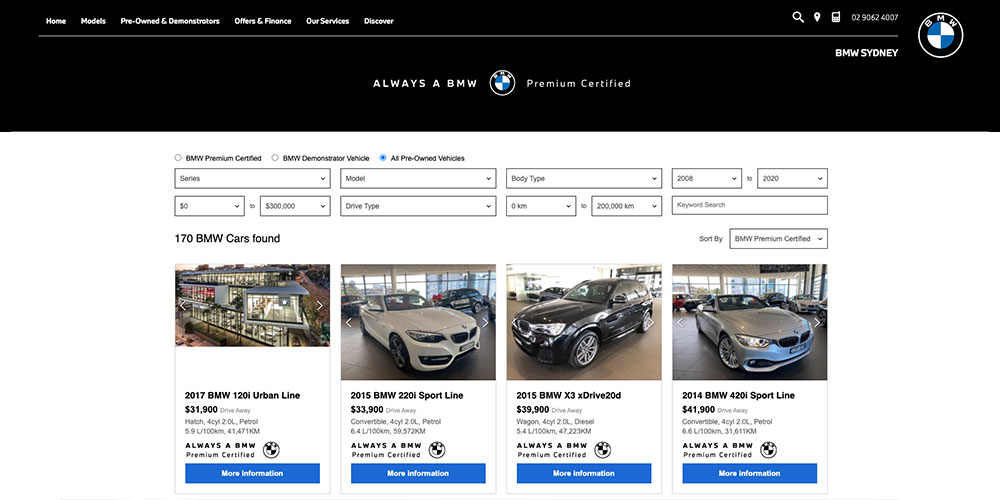The image depicts a detailed webpage interface for a BMW dealership, with a sleek black header and various navigation tabs at the top. The tabs are labeled "Home," "Models," "Pre-Owned and Demonstrators," "Offers and Finance," "Our Services," and "Discover." On the right side of the header, there are icons for search, location, and smartphone, followed by the contact number 02-906-24007. The BMW logo, which features a white-bordered circle with a black background and the letters BMW in white, is also present. Inside the logo, there is a segmented circle with alternating blue and white quadrants. 

Below the header, in the center, bold white text displays "Always BMW" alongside the BMW logo. Next to it, "Premium Certified" is noted in regular white text. The main content area features several rectangular sections organized in rows. On the left, a grey circle labeled "BMW Premium Certified" in bold black text is clickable. Following this are options for "BMW Demonstrator Vehicle" and the selected "All Pre-Owned Vehicles," highlighted in blue.

A series of dropdown menus follow for filtering results by "Series," "Model," "Body Type," "Year Range (2008 - 2020)," "Price Range ($0 - $300,000)," "Drive Type," "Kilometer Range (0 - 200,000 km)," and "Keyword Search." On the left-hand side, bold black text states "170 BMW cars found," while on the right, there is a "Sort By" dropdown menu next to "BMW Premium Certified."

The primary section showcases a front view of the BMW dealership building, illuminated with white and yellow lights and surrounded by trees and flowers. Listings for various cars follow:

- **2017 BMW 120i Urban Line** - Priced at $31,900, with "Always BMW" in bold black and "Premium Certified" in black beneath it. Each listing features a clickable dark blue button labeled "More Information."
- **2015 BMW 2020i Sportline** - Priced at $33,900, a silver car with white accents is displayed with red and black cars in the background.
- **2015 BMW X3 xDrive 20d** - An SUV in black, priced at $39,000.
- **2014 BMW 420i Sportline** - A dark gray car listed at $41,900.

Each vehicle entry on the page features consistent branding elements, ensuring a uniform presentation across the site.